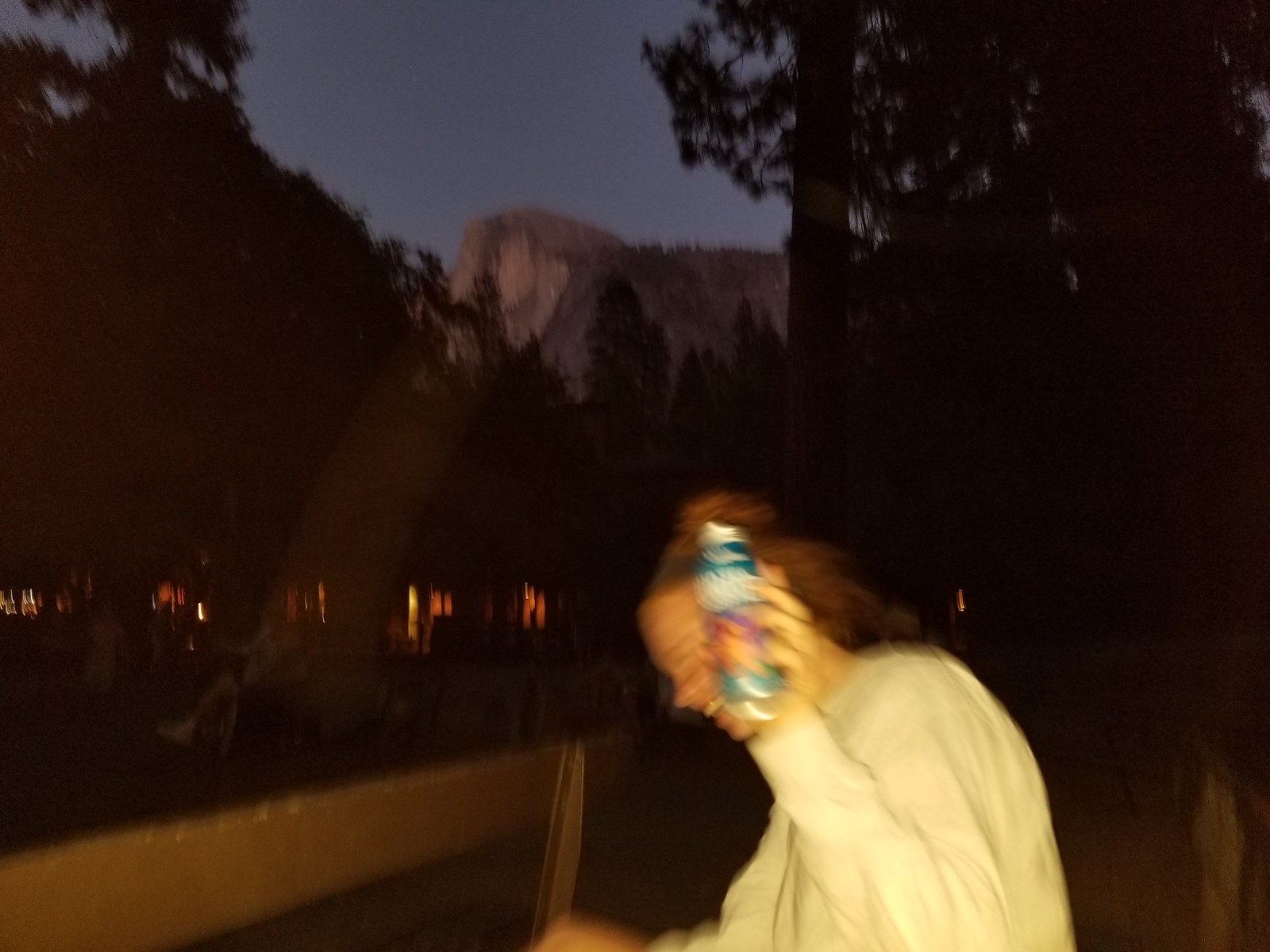In this extremely blurry and dark photograph, captured likely at twilight with an older camera, a young woman aged between 18 to 22 is seen laughing heartily, her body in motion. Her reddish-blonde hair is partially pulled into a high ponytail, while the rest cascades down. She is dressed in a long-sleeved white shirt or sweatshirt, and in her left hand, she holds a turquoise, white, and pink can, presumably a beverage. The scene unfolds outdoors, possibly in a park-like area, with a wooden fence in the foreground and the faint outline of a park bench nearby. In the dim background, pine trees and ponderosa pines rise up, and a distant mountain summit stands against an indigo sky transitioning to night. Scattered people seated on chairs and softly illuminated buildings enhance the setting’s ambiance, while the dark, cloudless, and starless sky overhead reinforces the dusk or nighttime atmosphere.